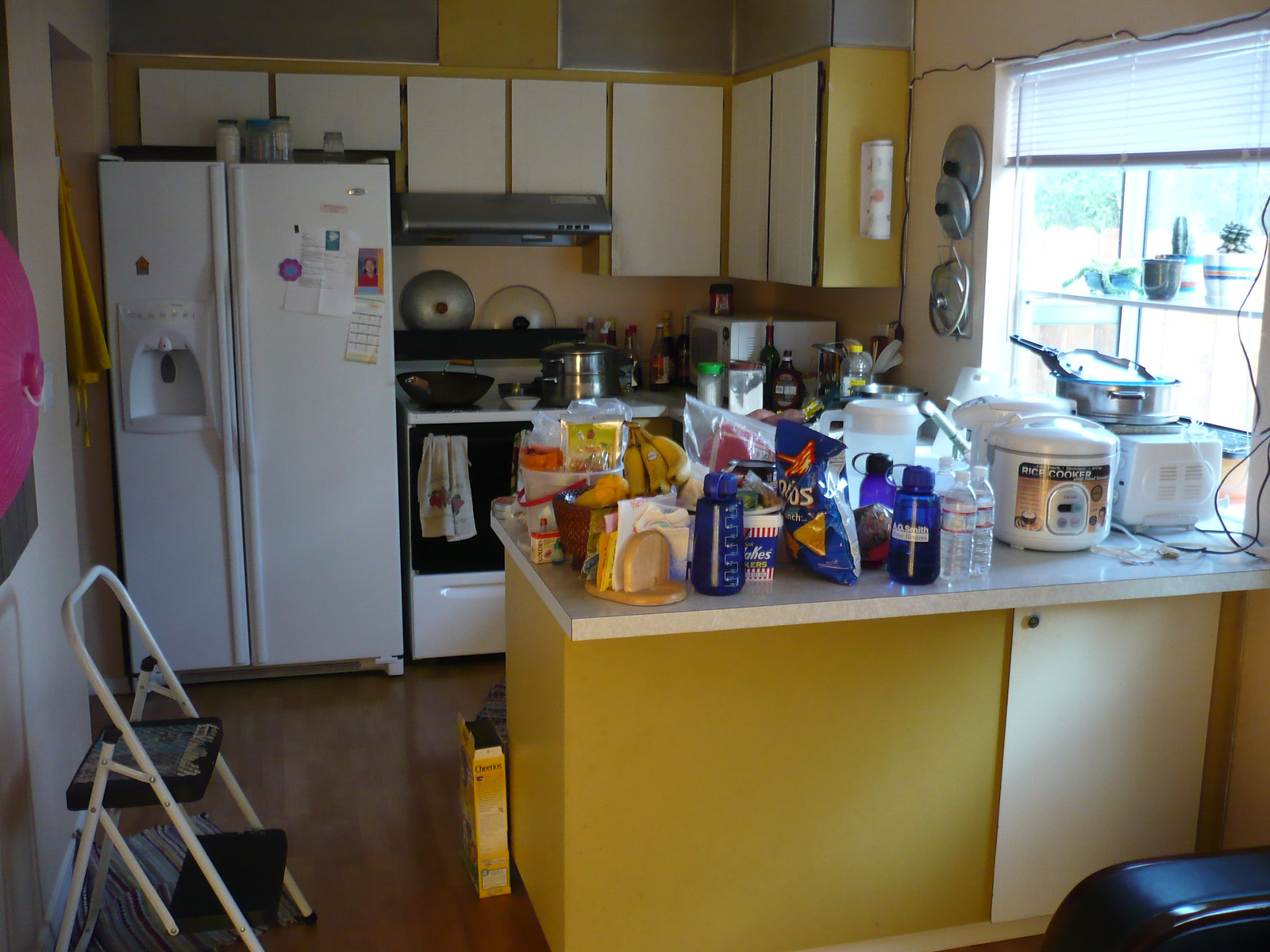The photograph showcases a kitchen featuring a prominent side-by-side refrigerator in the upper left corner, exuding a pristine white finish. Above the refrigerator, 90s-style cream-colored cabinets line the wall, extending to the right over a sleek stainless steel hood range. Below the hood sits a white stove, distinguished by a black oven door and a matching black control panel at the top, with a couple of potlets resting behind it. More cream-colored cabinets continue above the stove and around the corner, transitioning to the adjacent wall with two additional cabinets. The white countertops are cluttered with a variety of items, resembling a recent grocery haul. Among the items are a bag of Cool Ranch Doritos, bottled water, bananas, and various indistinguishable containers. Additional details include a water bottle, a napkin holder, and a dish towel draped over the stove handle. A practical two-step step ladder is positioned in the bottom left of the image, completing the scene.